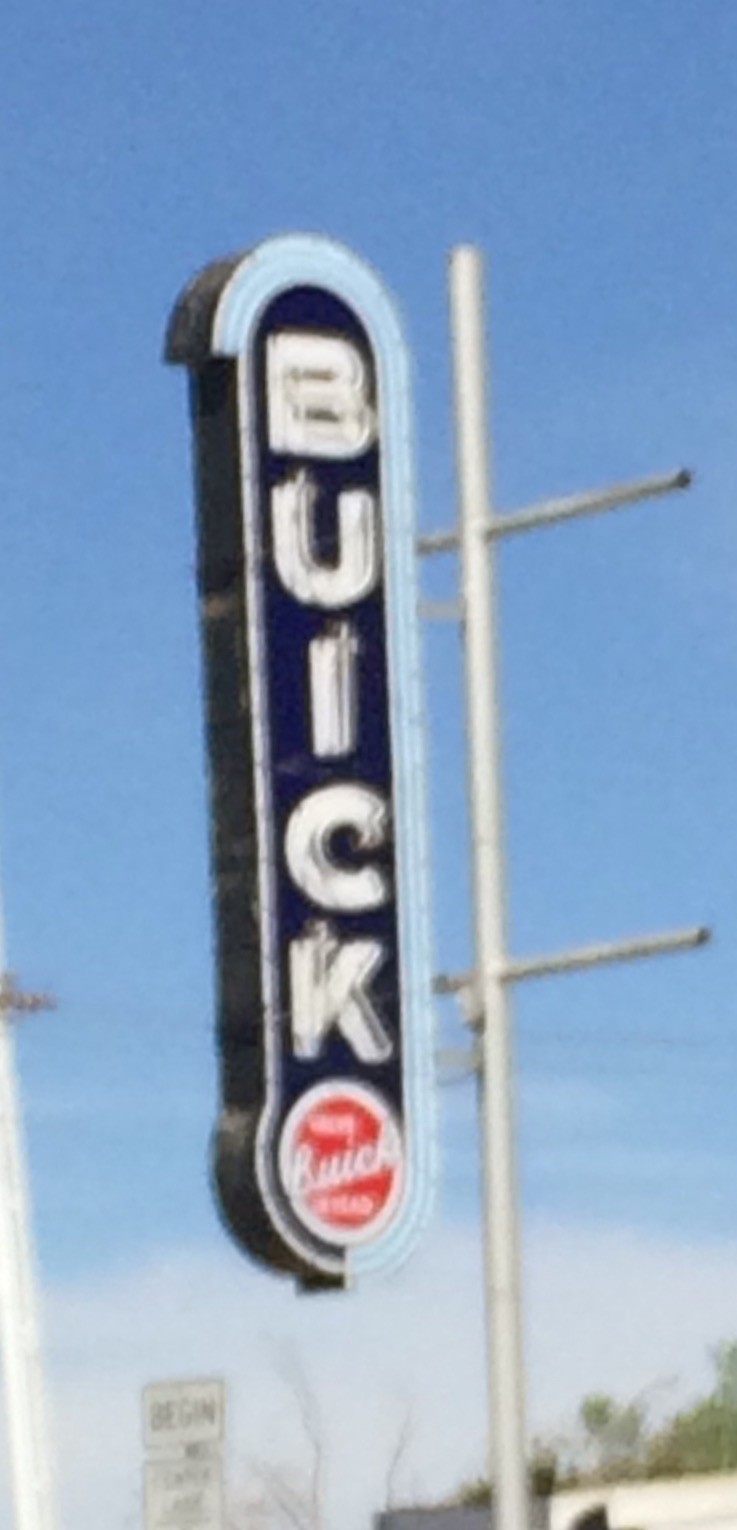A vertically aligned sign spells out "BUICK" with each letter stacked one beneath the other, creating a columnar arrangement. Below the letters, there is a red circle containing the word "Tribe." The image appears to be cropped tightly to emphasize the sign, minimizing surrounding elements and drawing the viewer's attention directly to the vertical alignment of the letters and the red circle at the bottom. There are other objects and details present around the sign, but they are not visible in the cropped frame.